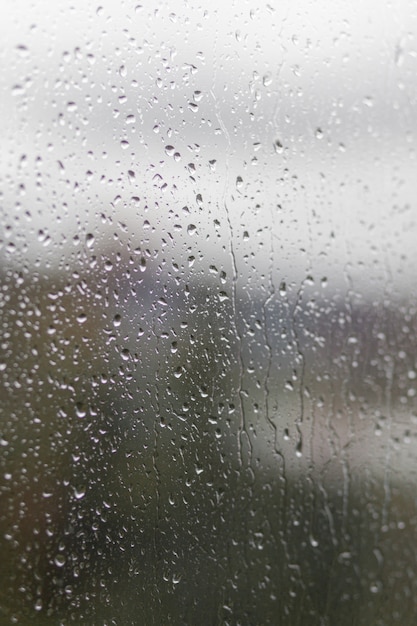This photograph captures a rainy scene from inside a building, looking out through a window pane covered in raindrops. The water droplets, some stationary and others sliding down, obscure the view of the outside. The background behind the window is blurred, dominated by a gray sky with lighter patches suggesting a foggy day. Muted green and brown foliage is partially visible through the haze, providing a natural contrast of colors. The lower part of the scene appears darker, transitioning from dark gray to black, while streaks of green add more color variation. To the right, a lighter, indistinct mass adds an additional element of intrigue to the blurry backdrop, enhancing the overall atmosphere of a rainy day viewed from the safety and warmth of indoors.